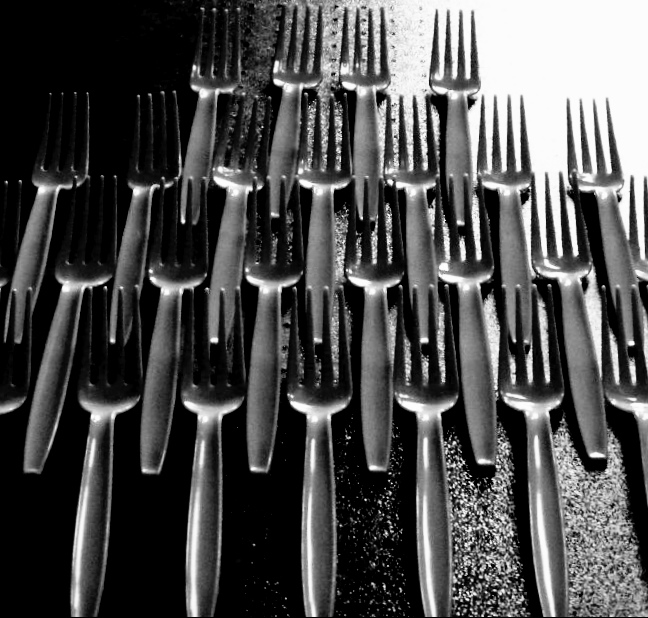This black-and-white photograph depicts a neatly arranged series of plastic forks, possibly resembling a work of art. The forks are laid out on a dark background, organized in staggered rows that interlock with one another to create a pyramid-like formation. Precisely, the bottom row consists of five forks, the second row six, the third seven, and the topmost row contains four forks, cumulatively around 22 forks. Each fork has short tines and handles with concave surfaces, which may appear either hollowed-out or raised due to the monochromatic color scheme. The lighting intensifies the reflective quality of the forks, particularly noticeable in the upper right corner where a bright patch of light contrasts with the primarily black backdrop on the left. The interplay of light and shadow emphasizes the delicate, perhaps flimsy nature of the forks, suggesting they are made of plastic, although their metallic-like sheen leaves room for ambiguity.